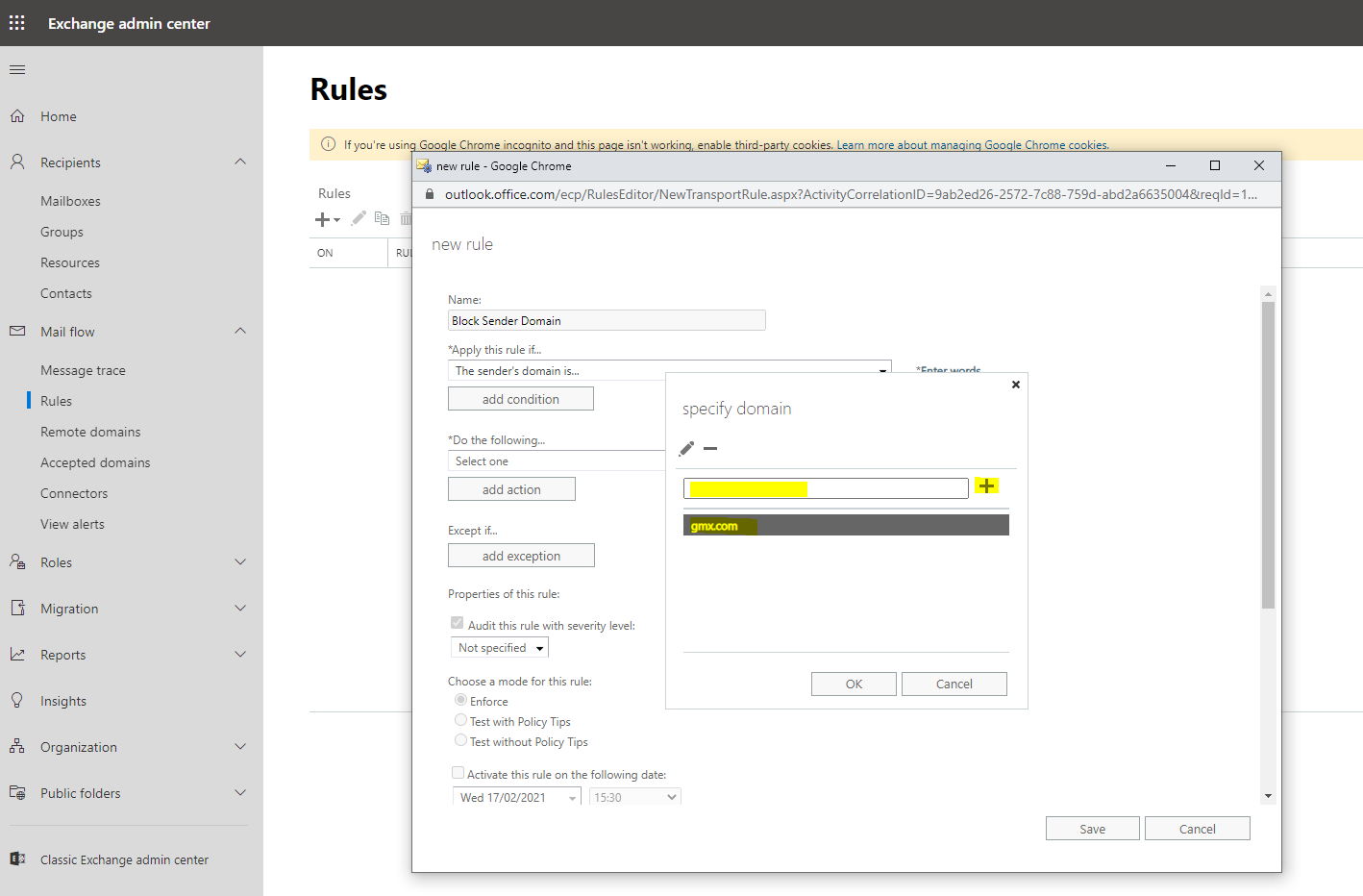This image depicts the Exchange Admin Center interface of administrative software. On the upper left-hand side, the title "Exchange Admin Center" is prominently displayed. The layout features a vertical navigation menu on the left side of the screen, comprising various admin categories: starting with Home, followed by Recipients, Mailboxes, Groups, Resources, Contacts, Mail Flow, Message Trace, Roles, Migration, Reports, Insights, Organization, and Public Folders.

A popup window titled "New Rule for Google Chrome" is open, showing a process taking place within the interface. Inside this popup, there is another smaller window titled "Specified Domain." Highlighted in yellow within this smaller window is an input box where the domain "gmc.com" is being added. The highlight emphasizes the current focus of this administrative task, suggesting an emphasis on configuring rules associated with this domain.